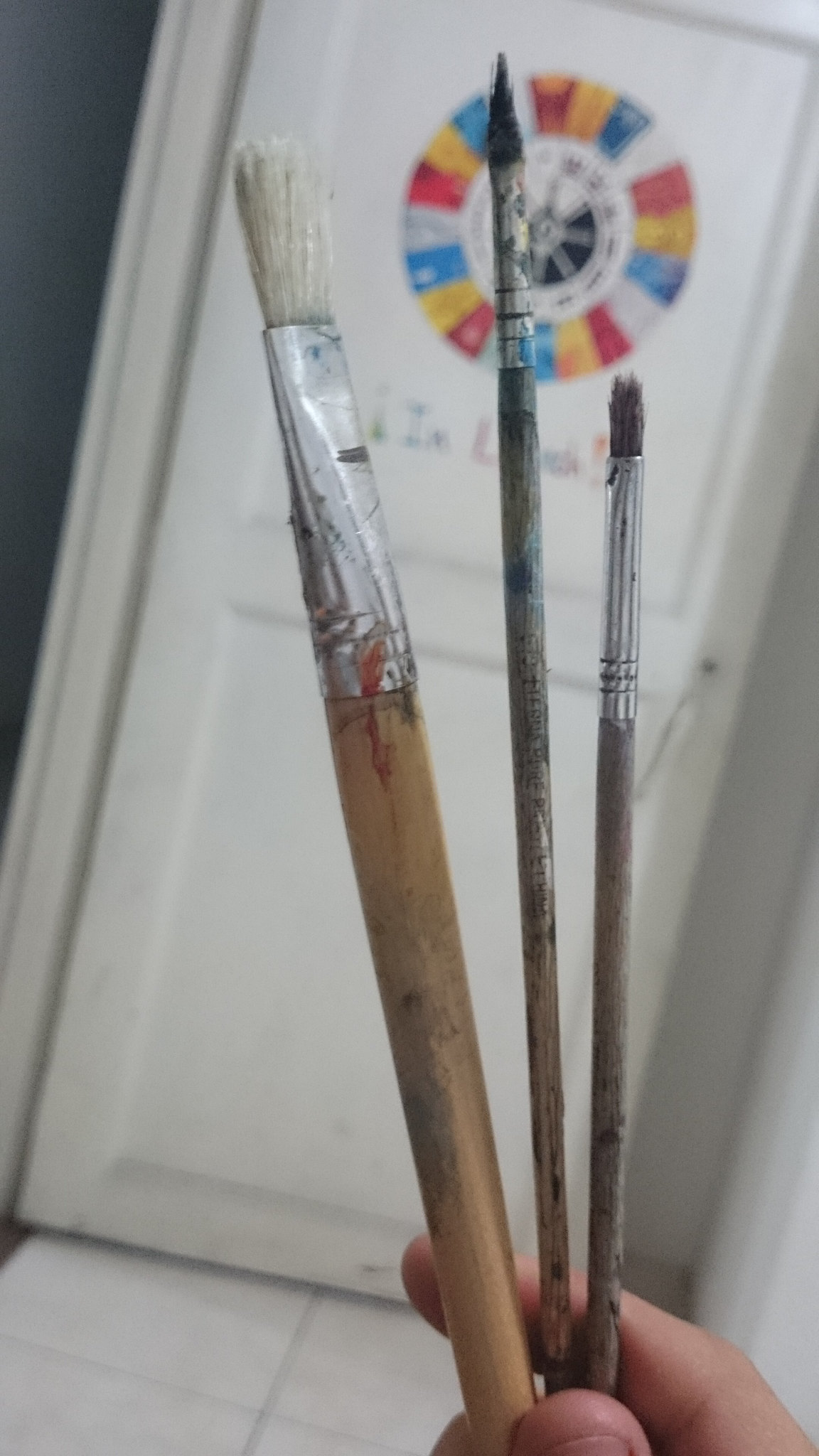In the image, a person's fingers, possibly of Caucasian descent with short nails, hold up three different paintbrushes in front of a white door that has a colorful, blurred poster on it. The floor beneath appears to be white, possibly tiled. The paintbrush on the left is large and wide, with a white brush and a silver metal ferrule that narrows towards the wooden handle. The middle brush is long and thin, also featuring a metal binding and a pointed black bristle tip. The rightmost brush is the shortest and smallest, with a square-shaped black bristle and a metal ferrule. All the brushes show signs of use, indicating they are likely employed for artistic painting.